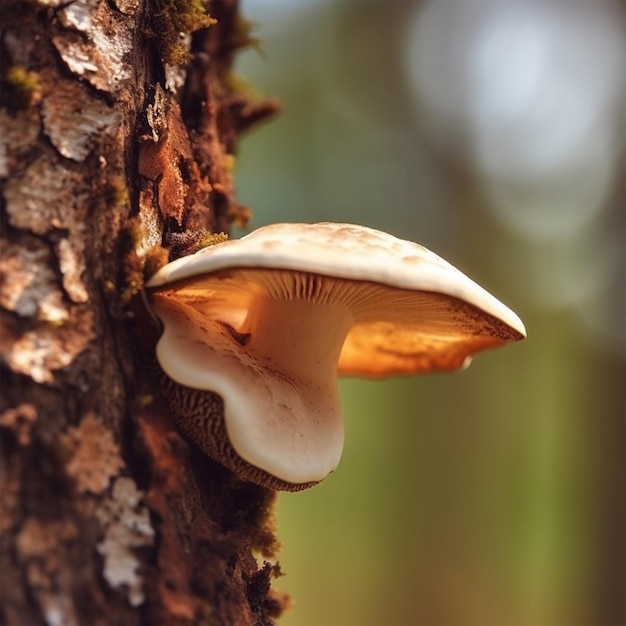This macro photograph captures a single toadstool emerging from the reddish-brown bark of a tree. The close-up detail highlights the thick, short, creamy white stem of the mushroom, which appears almost rubbery. The cap of the toadstool transitions from a standard creamy white with brown flecks on top to an orangish-yellow glow underneath, as light filters through, giving it a translucent, almost glowing appearance. The bark, characterized by its flaking texture and shades of brown ranging from deep hues to lighter tones, contrasts against the blurred green and white background, creating a soft, indistinct backdrop that emphasizes the intricate details of the mushroom and tree bark. The overall scene evokes the imagery of a toasted marshmallow, particularly where the mushroom cap appears almost melted over the tree bark.